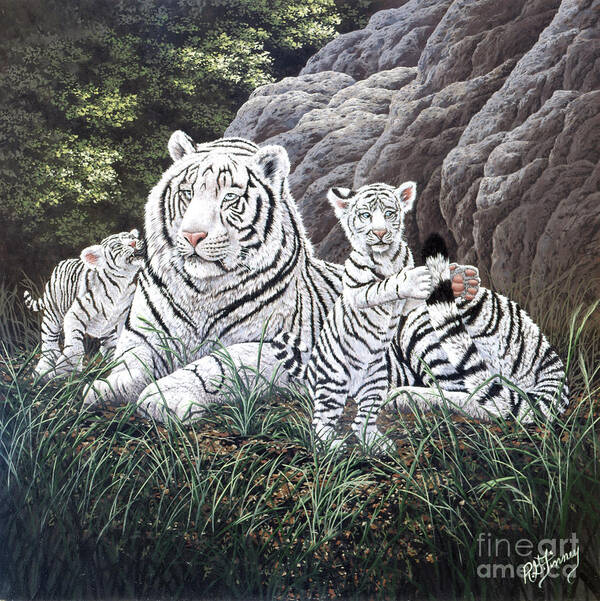This detailed artistic piece depicts a majestic white tiger reclining from right to left, with two playful cubs by her side, all adorned with striking black stripes. The scene is set against a composite background combining a photograph of a rugged, gray rocky hill and a grove of trees on the left. The foreground features scattered shoots of tall grass. The tiger, slightly facing left, anchors the composition. The cub on the left of the image (the tiger's right side) is baring its teeth and standing on all fours. The other cub, positioned on the right (the tiger's left side), is standing on its hind legs, engaging with the mother's tail between its paws. The artistry blends seamlessly with the photographic elements, creating a lifelike yet imaginative scene. The image is signed in the lower right corner with "Fine Art America" and an artist signature that appears to be "RG Timmy" or "Jimmy."